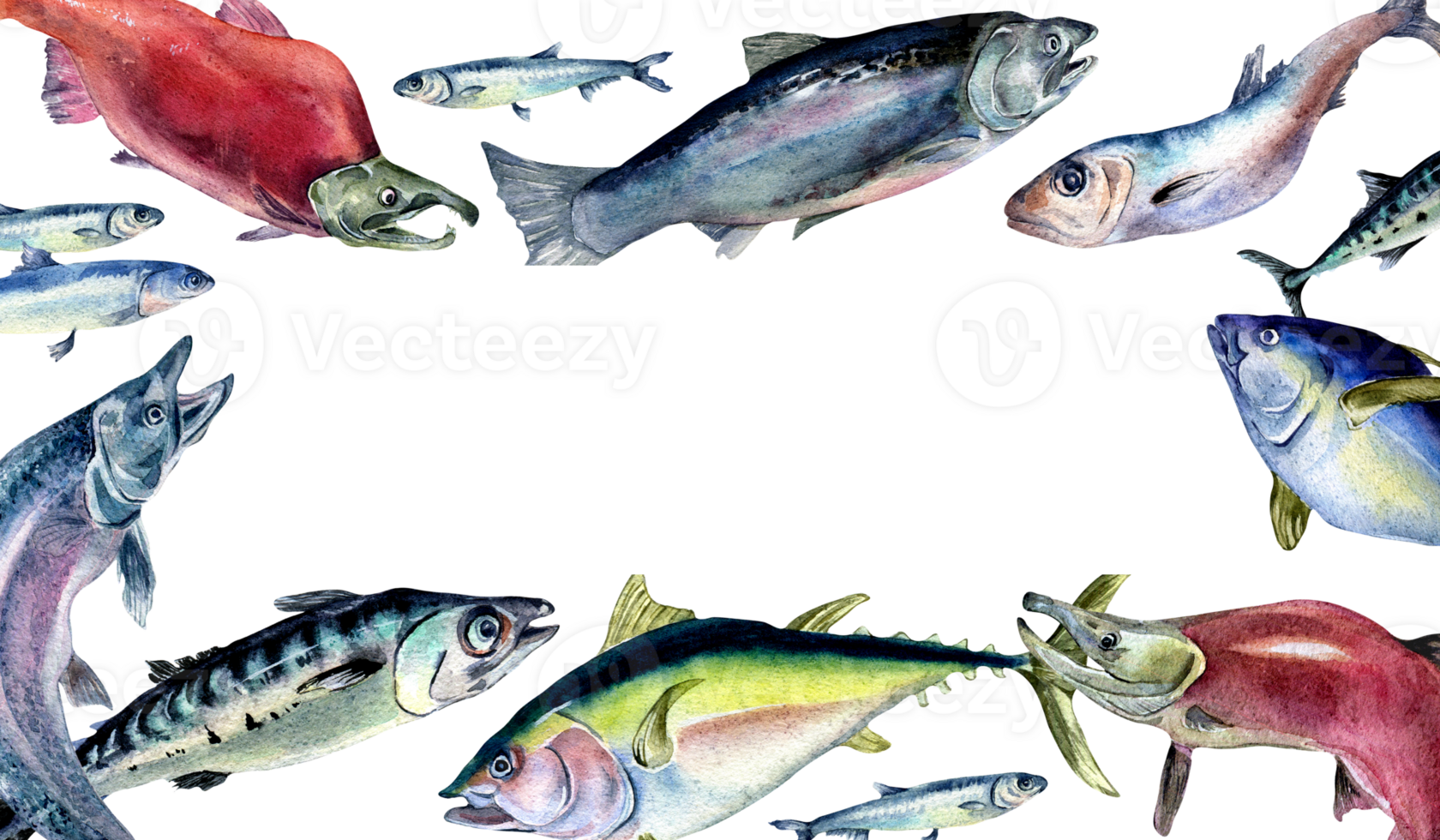This detailed color illustration against a white background depicts a variety of fish species, each artistically rendered with a cartoonish and almost animated style. The fish vary greatly in color and size, creating a lively and diverse scene reminiscent of tropical waters.

Prominently featured is a bright mahi-mahi at the bottom center, easily identifiable by its characteristic black back and yellow stripe, alongside a greenish hue on its belly. Adjacent are several smaller fish, five in total, contributing to the abundant diversity of the composition. Among these smaller fish is a silver-gray sardine and a salmon, identifiable by its red body and distinctive beak-like snout.

In the upper section, there appears to be tuna, notable for their streamlined bodies, including one with a striking blue and yellow palette. Additional red fish with notably ugly, open snouts further add to the varied visual texture. There's also a mention of a bluefin tuna and a barracuda, integrating a sense of both familiar and exotic marine life.

Arranged thoughtfully, the fish seem to swim in a square pattern, enhancing the artistic quality of the drawing. The illustration bears the silhouette of a text, "Vect TZ," possibly hinting at the artist or the artwork's title, accompanied by a cursive "V" symbol. This vibrant and meticulous representation captures the viewer's attention with its rich detail and colorful composition.